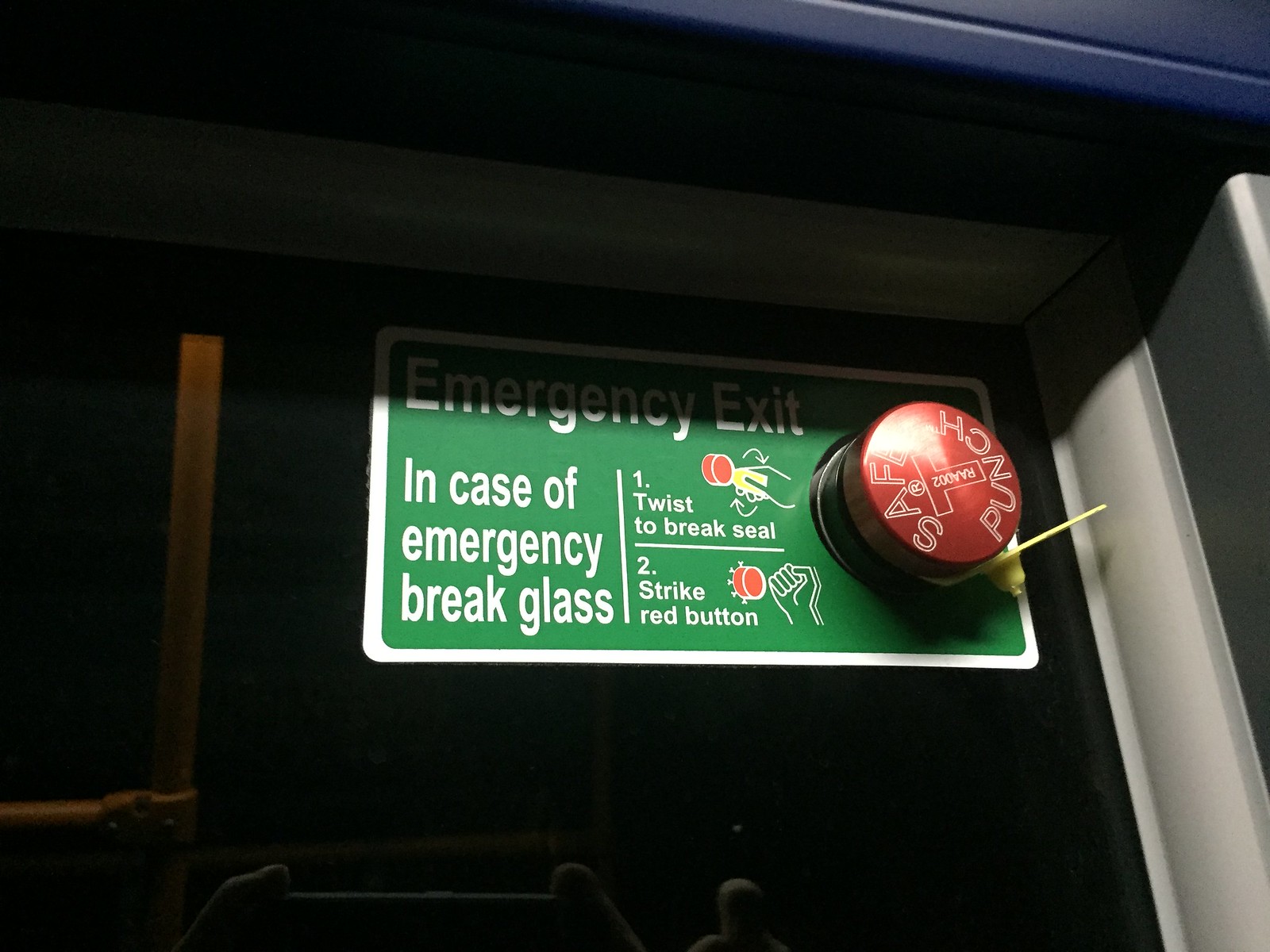The image depicts an emergency exit sign with detailed instructions for use. The green rectangular plaque displays "Emergency Exit" in bold white letters. Beneath this, it reads "In case of emergency break glass" although the glass isn't visible in the frame, suggesting it might be behind the sign. To the right, step-by-step instructions adorn the right half of the plaque. Step one instructs "Twist to break seal," accompanied by an image of a hand twisting to break a seal, highlighting a yellow tab near a large red button. Step two reads "Strike red button," illustrated with a fist striking the button. The button prominently juts out from the plaque and is labeled "Safe Punch" in white lettering. The entire setup is against a black window-like background, with shadows hinting at a nearby doorframe affecting the light.